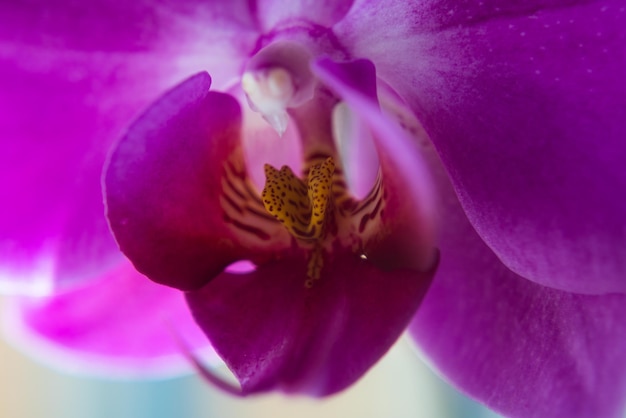This image presents an extreme close-up of a beautifully detailed flower. The intricate petals showcase a gradient starting with a vibrant purple on the edges, transitioning to a lighter, almost white hue near the center. The central portion of the flower is highlighted by a unique combination of patterns—dots, and stripes reminiscent of zebra stripes and cheetah prints—adding to its exotic appearance. Protruding from the center is a prominent purple stem and a distinct white area that almost appears to harbor a pearl-like object. This middle area also features a striking yellow section adorned with black polka dots, emphasizing the complexity of the flower's anatomy. The flower appears to be angled downward, directing its focus toward the bottom of the image. The blurred background, featuring shades of tan and blue, enhances the flower's vivid details by creating a contrasting, out-of-focus backdrop.